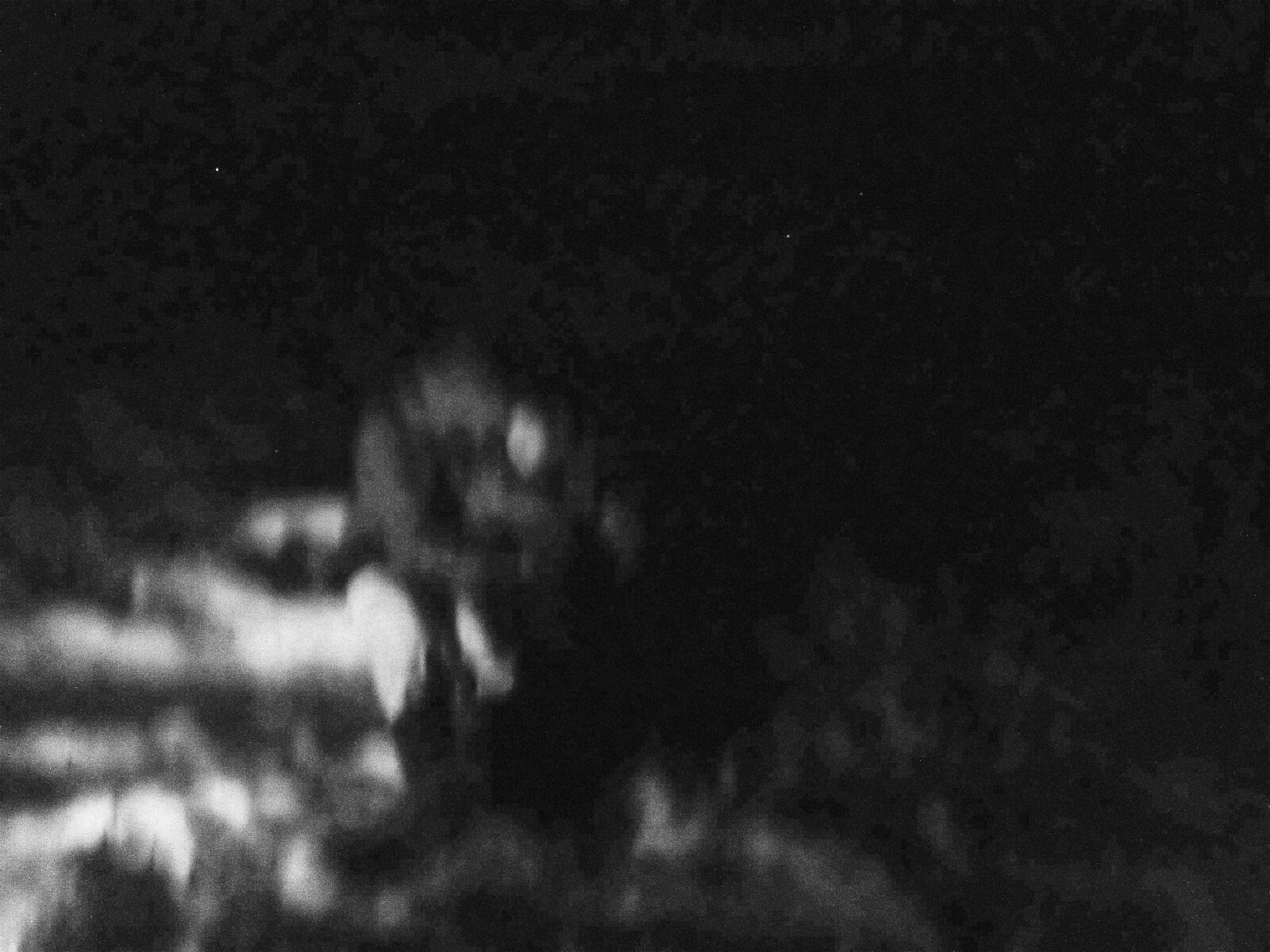The photograph in question is a very dark, grainy, and out-of-focus black-and-white image. Spanning from the top left to the bottom right corner, it is predominantly black, interspersed with various blurred gray and white sections. There is an identifiable portion on the bottom left side of the image where a white blur is connected to a gray blur, which in turn has white dots at the top and bottom. Underneath these white dots, there is a gradient of gray blurs that fade into the darker background.

Amid the indistinct blurs, one can faintly discern the outlines of two figures, possibly a man and a woman, who appear to be sitting together outside in the grass. The man seems to be holding the woman close, though his face is not visible. The outline of the woman's face is slightly more distinguishable. They seem to be alone in the dark, with the outline of what might be a car visible behind them, suggesting they could have parked and stepped out for some personal time.

While the exposure issues and blur impede absolute clarity, the lighting within the photo highlights certain features, casting reflections that provide subtle hints of the scene. There is no text present in the image, indicating that it might be a photographic print that developed with significant imperfections.